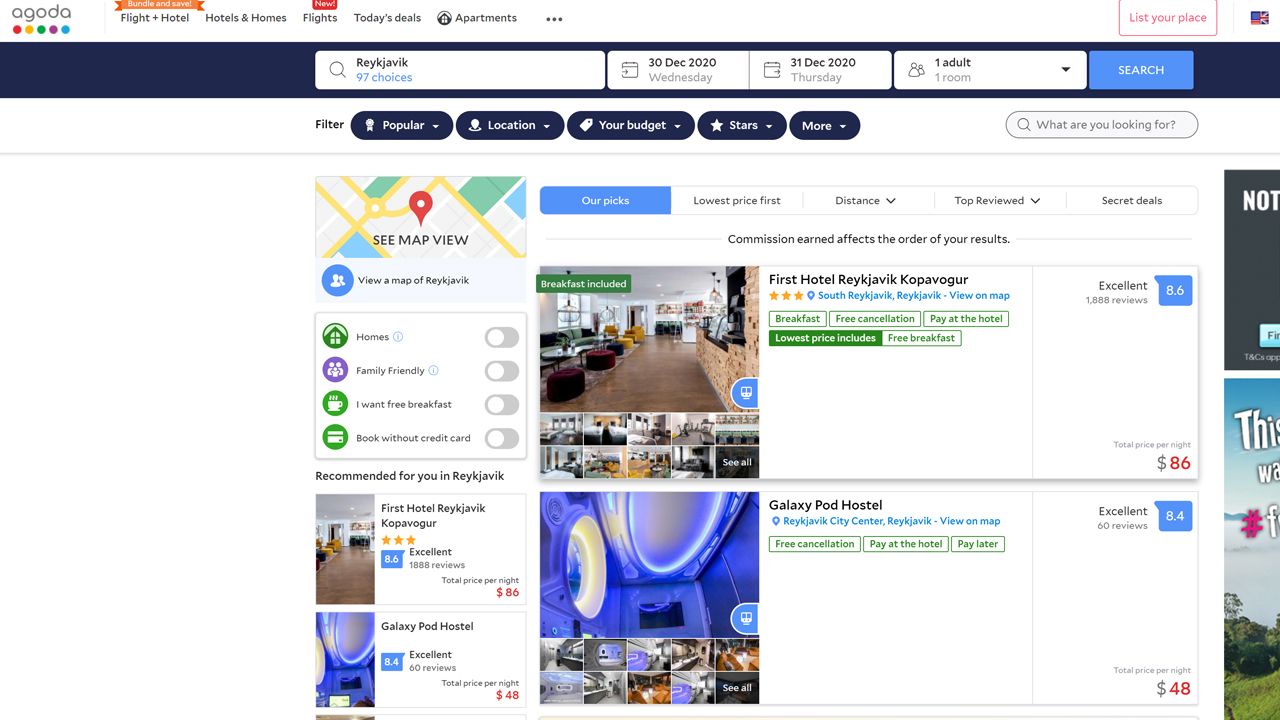**Caption:**

A detailed screenshot of a travel website, specifically Agoda, showcasing various booking options for a trip to Reykjavik. The header features Agoda’s logo and navigation tabs for flights plus hotel, hotels and homes, flights, today’s deals, and apartments. The search bar displays "Reykjavik, 97 choices" with date selections for December 30, 2020 (Wednesday), and December 31, 2020 (Thursday). The search criteria indicate one adult and one room.

Below the search bar, filters are available for popular choices, location, budget, star ratings, and more. An image of a map is accompanied by options to view the location of Reykjavik hotels on the map. Below this map view, filter options include homes, family-friendly stays, free breakfast, and book without credit card, none of which are selected.

The main section reveals recommended hotels in Reykjavik. The first recommendation is the First Hotel Reykjavik Copenhagen, illustrated with an interior room photo and nightly pricing. Another option is the Galaxy Pod Hostel, also showcased with a price per night and its interior room image.

On the right-hand side, a highlighted tab titled "Our Picks" features the First Hotel Reykjavik Copenhagen, which has an excellent review score of 8.6, includes breakfast, and costs $86 per night. Another highlighted option in this section is the Galaxy Pod Hostel, priced at $48 per night, shown with a large image of its interior.

Overall, the screenshot provides comprehensive details to aid travelers in making an informed decision for their stay in Reykjavik.